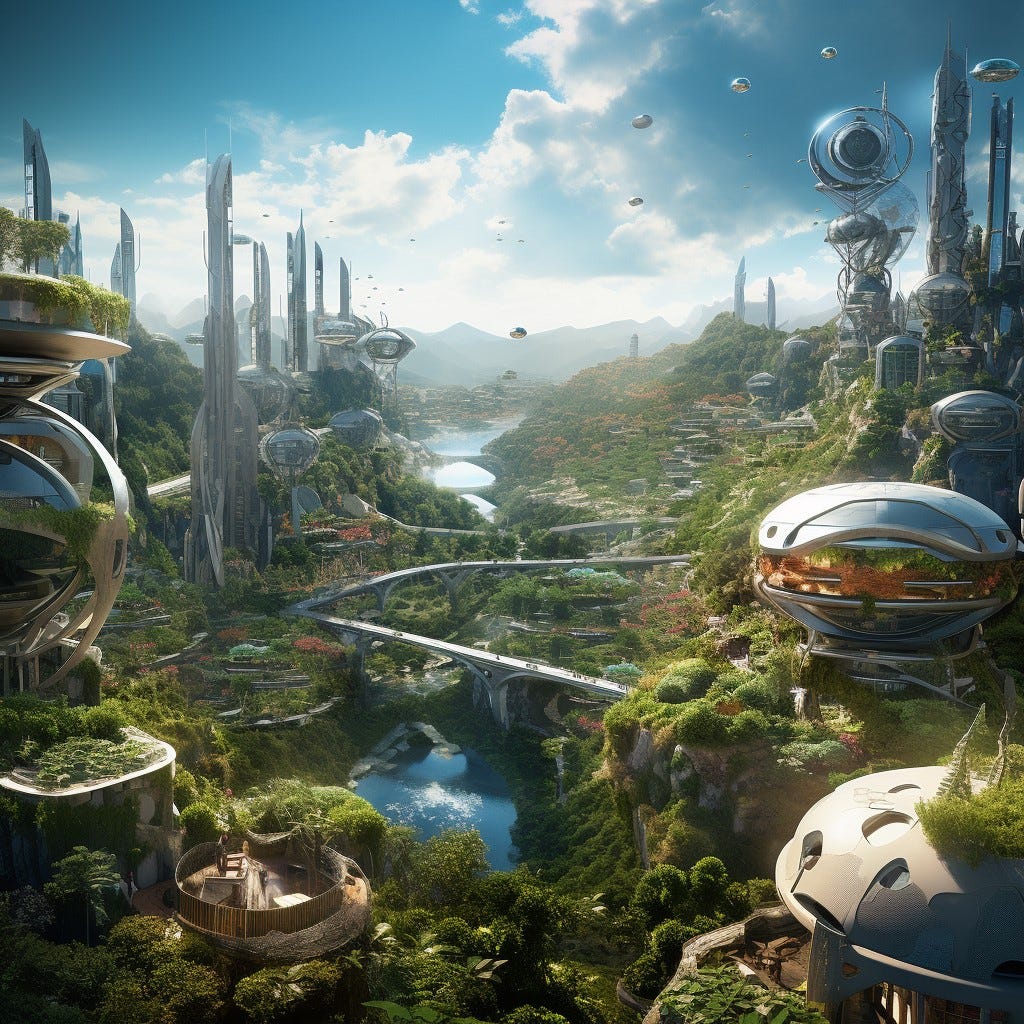The image is a detailed 3D rendering of a futuristic city set within a square frame. Dominating the skyline are an array of futuristic buildings, many of which are tall, silver, and thin, while others have a unique, oval, UFO-like shape. Some of these oval structures serve as homes, blending seamlessly into the innovative urban landscape. The city is nestled in a lush environment filled with abundant greenery, including green grass, trees, bushes, and even patches of red flowering plants.

The setting features a bright blue sky dotted with white, puffy clouds, enhancing the vivid color palette of the scene. Amidst the skyscrapers, there are also aerial spacecrafts floating in the sky, resembling metallic, hamburger-shaped crafts. A significant element of the image is its intricate roadway system, which includes elevated highways supported by massive girders and beams, stretching across a vibrant blue river flowing through a valley in the lower part of the image. The clarity and vibrant lighting of this highly detailed concept art evoke a vivid and imaginative vision of a sci-fi metropolis.